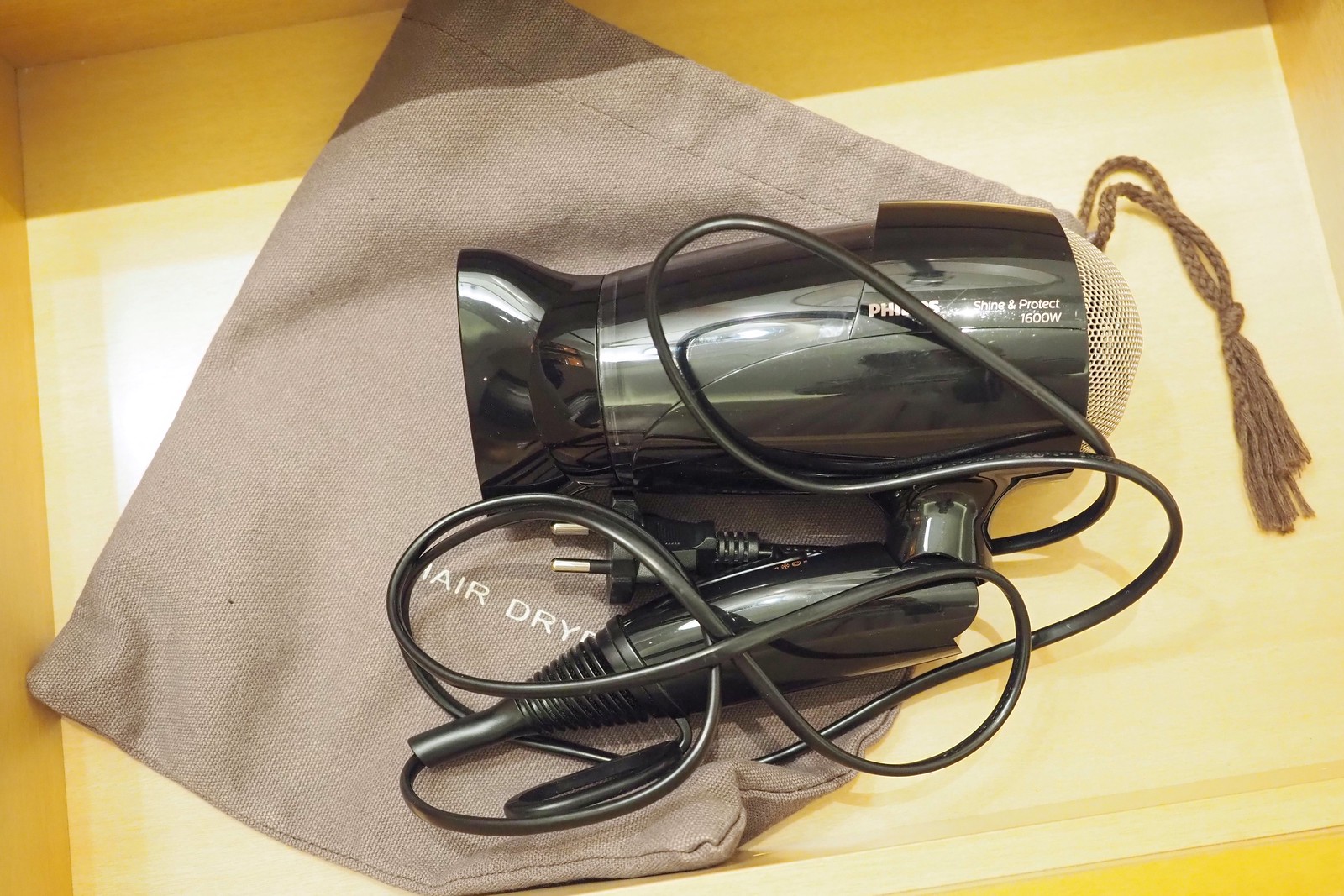The photograph features a compact, portable Philips hair dryer, primarily black with possible hints of green or dark gray nuances. The close-up shot showcases the hairdryer laying on its corresponding brown canvas travel bag, which has a drawstring top. The hairdryer, which appears to be designed for travel, has a folding handle for easy packing. It is equipped with a long, black power cord, approximately 3 to 4 feet in length, wrapped around the device. Notably, the hair dryer's surface bears white text that reads "Project 1500W" or "Protect 1600W," indicating its power capacity. Additionally, the hair dyer also involves a wide black nozzle and a silver mesh shield at the air intake point. The entire setup is placed inside a yellow box, suggesting convenient storage and portability for travel purposes.